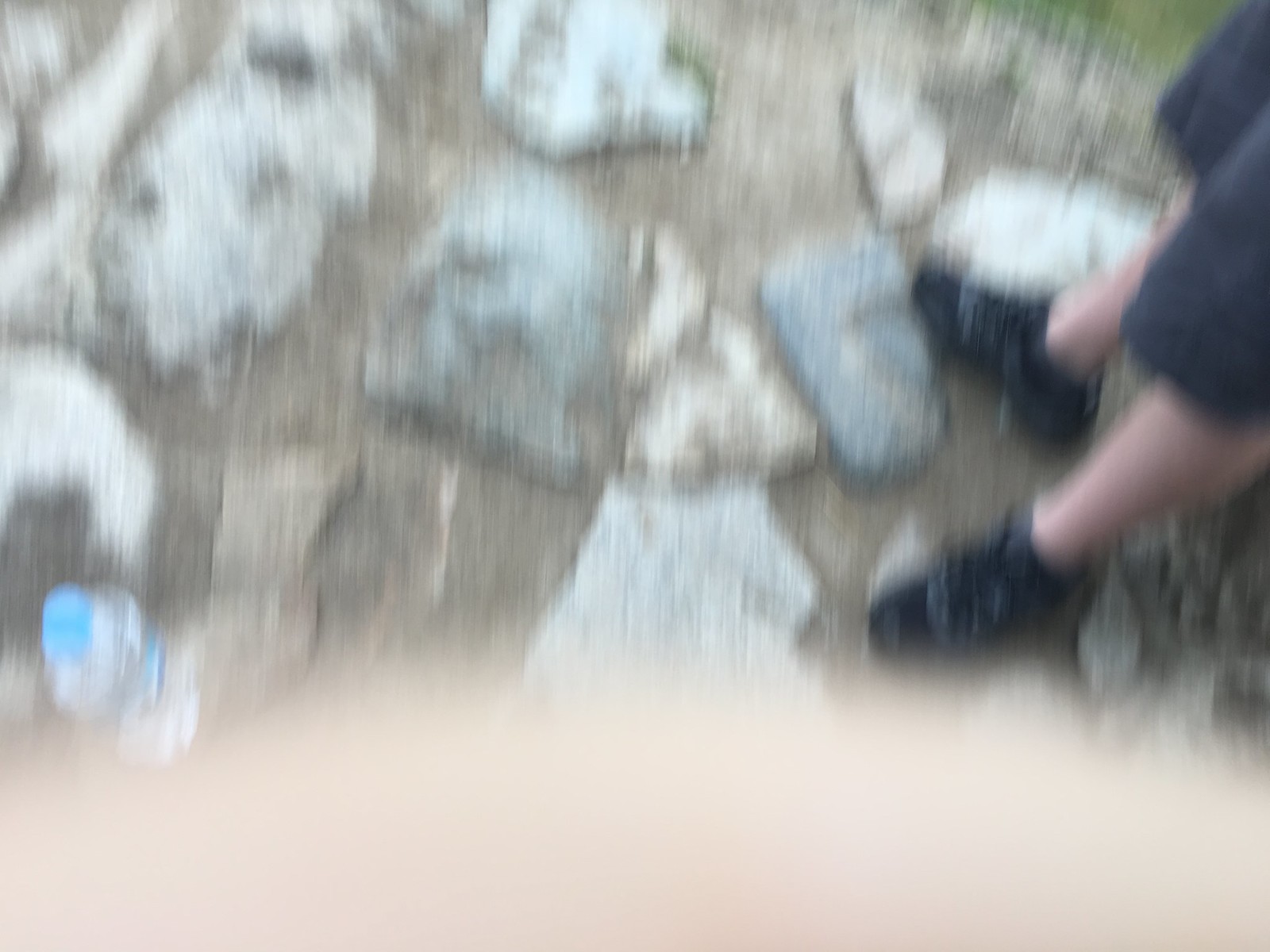The image is a low-quality, blurry photograph of the ground, possibly taken unintentionally. The bottom portion of the image is partially obscured by a tan or pink hazy object, likely a finger overlapping the lens. The ground consists of dirt interspersed with rugged, natural stone stepping stones in various shades of gray and tan, suggesting a stone path or walkway. In the bottom left corner, there is a plastic water bottle with a blue cap. On the right side of the image, the lower half of a person wearing black shorts and black shoes is visible. In the background, a sliver of a grassy field can be seen.